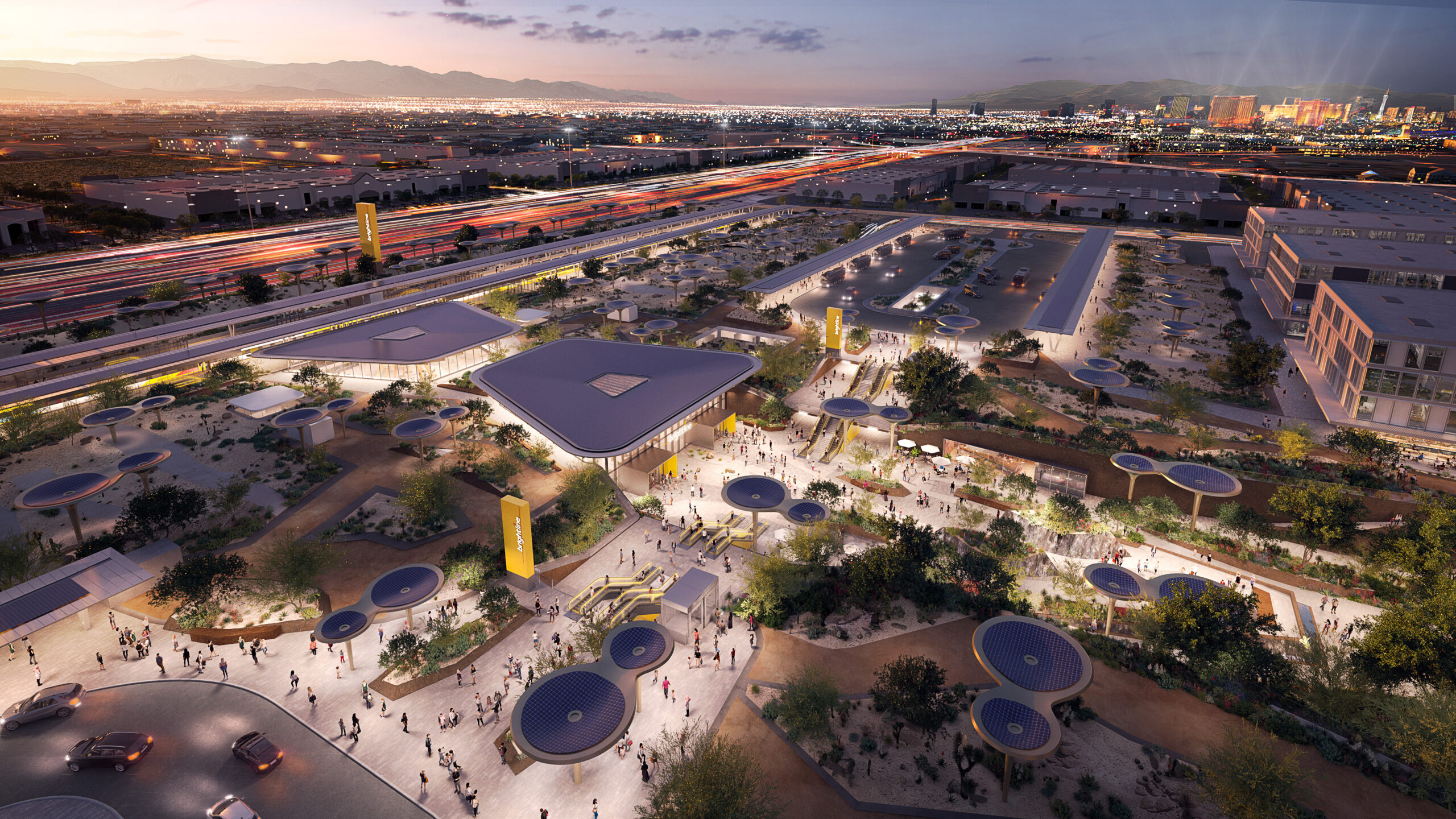The image is an aerial photograph taken from a high vantage point during the evening or early morning, capturing a broad, illuminated landscape that might depict a college campus or an urban outdoor theme park. The area is bustling with people and features large shaded spaces that resemble speaker-shaped parasols. The grounds are filled with various buildings, walking paths, and roads, all brightly lit. Large yellow signs with white writing stand out prominently. In the distance, the cityscape extends to the horizon, flanked by mountains and a large body of water at the center. The sky is adorned with clouds, adding depth to the detailed panorama.